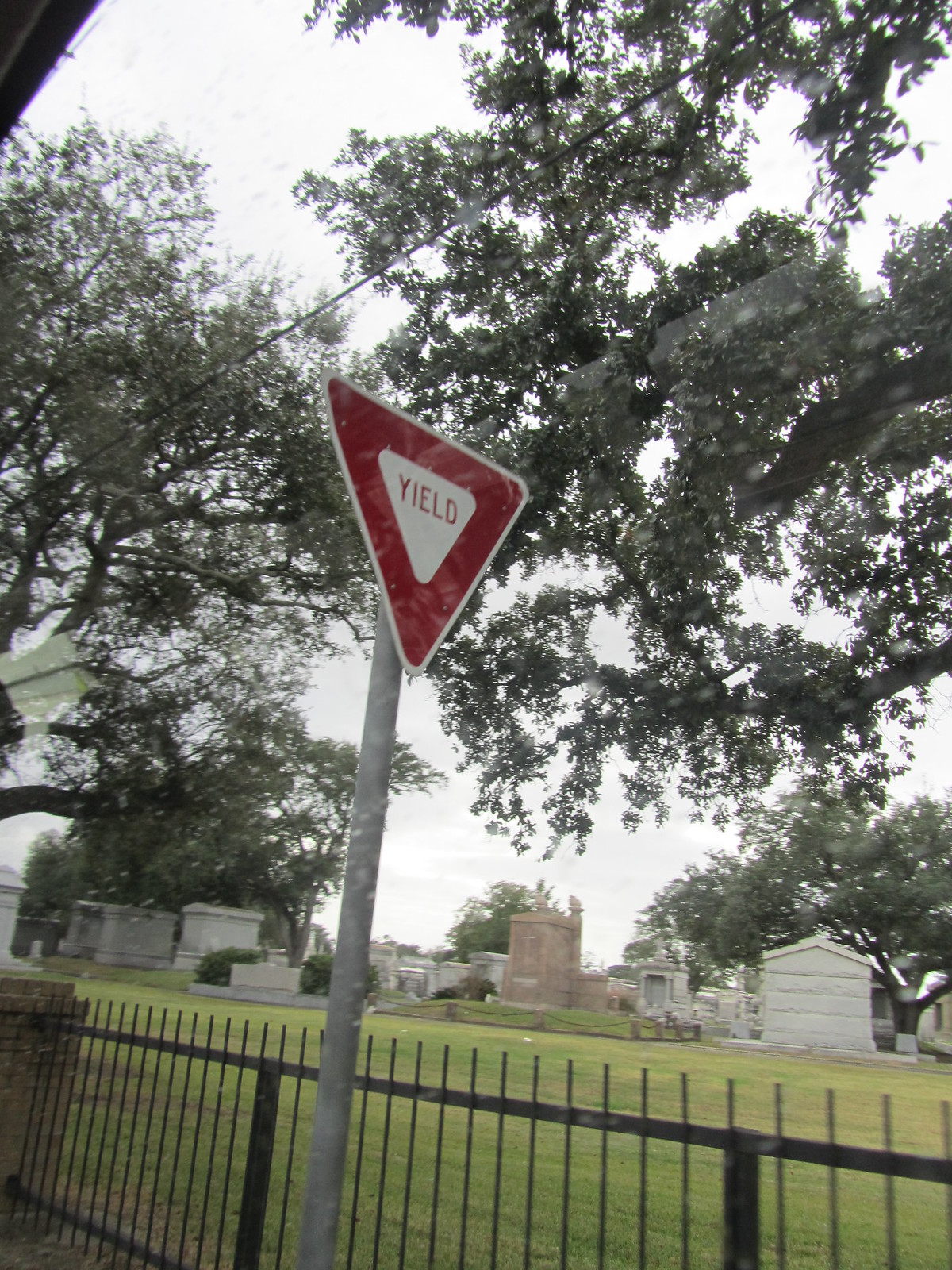The image captures an intricate view over a set of spiked metal railings overlooking a verdant park, which exudes a semi-sacred ambiance reminiscent of a churchyard. Among the lush greenery, large stone monuments rise prominently, while a chapel-like structure stands gracefully in the background. Sparse-leafed trees scatter around the foreground, their branches partially obscuring the scene beyond. A curious road sign—a red and white downward-pointing triangle that says "yield"—is positioned directly against the fence, creating an intriguing visual element. It remains ambiguous whether this sign is intended for pedestrians or motorists due to its placement right by the pavement.